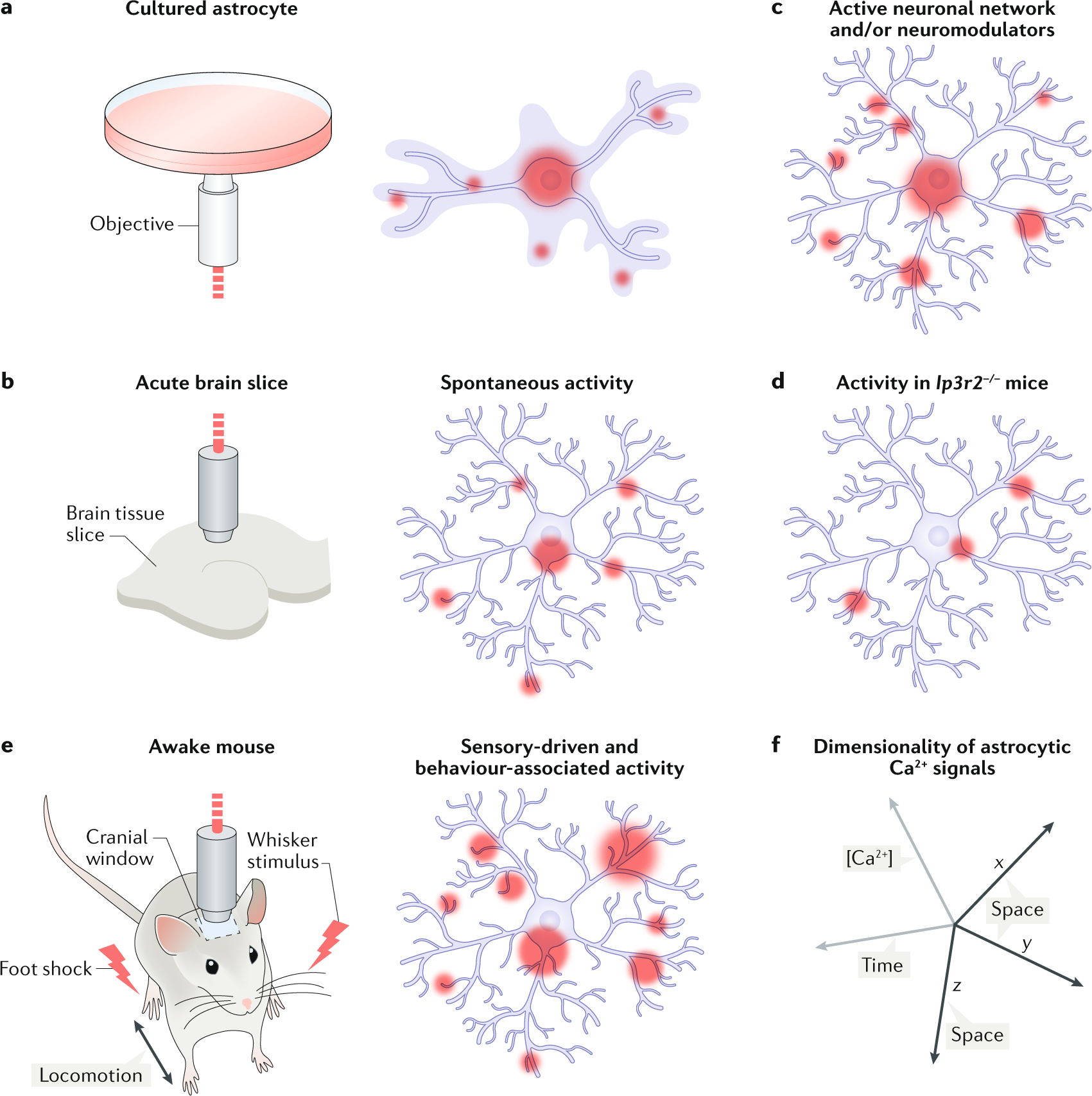The image is a detailed diagram consisting of nine illustrated images arranged in three columns and three rows, depicting various elements related to neuronal activity and astrocytic functions in the brain, likely of a mouse. 

In the top left corner, labeled "cultured astrocyte," there's a pink dish with a vertical column below it, indicating an examination setup. Adjacent to this, in the middle top position, is an illustration titled "objective," featuring a neural map with blue lines and interconnected structures marked by reddish dots, symbolizing an active area. The top right corner's image, labeled "active neuronal network and/or neuromodulators," shows a dendritic, coral-like structure with red hotspots, emphasizing active neural connections.

The second row begins with an image labeled "acute brain slice," illustrating brain tissue with a screw-like rod inserted, simulating in vitro analysis. In the middle position of this row, under the title "spontaneous activity," there's a depiction of a plant-like neural network with red dots, indicating active neural regions spontaneously firing. The right image in the second row, labeled "activity in IP3R2 mice," displays a similar network but with fewer red dots, highlighting specific neural activities in genetically modified mice.

The third row contains images related to live animal experiments. On the left, labeled "awake mouse," a drawing of a mouse shows a rod implanted in its head marked by red hotspots, indicating areas of neural activity. The middle image, also associated with sensory and behavioral responses, is marked "sensory driven and behavioral associated activity" and shows a neural network lit up by red dots. The bottom right image, labeled "dimensionality of astrocytic Ca2+ signals," presents a complex vector diagram resembling a snowflake, which illustrates the spatial and temporal dynamics of calcium signals within astrocytes across various dimensions.

Overall, the diagram lays out a comprehensive visual representation of different neuronal and astrocytic activities and experimental setups used to study these processes in mice.